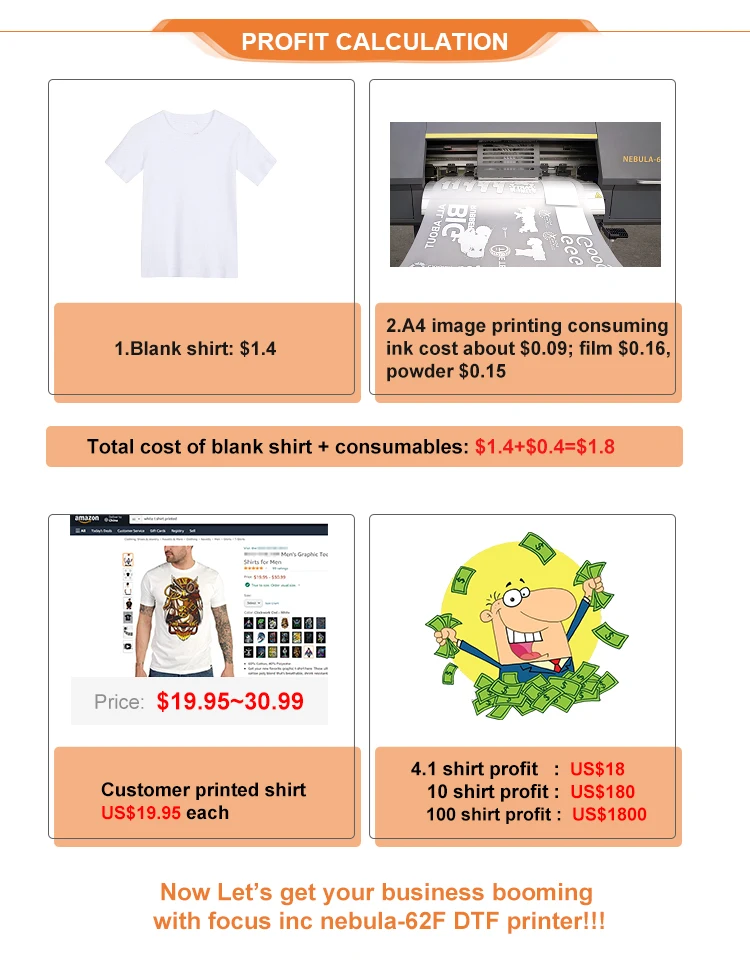**Caption:**
The image titled "Profit Calculation" features a sequence of detailed visual and textual information on calculating profit margins for printed t-shirts. At the top, "Profit Calculation" is written in orange, bold white lettering. The first section (number 1) displays a plain white t-shirt priced at $1.40. In the second section, the image outlines the costs associated with printing an image on the t-shirt: ink costing $0.09, film at $0.16, and powder at $0.15, summing up to $0.40. Combining the base cost of the shirt and the printing consumables, the total cost per printed t-shirt is $1.80.

Following this, the image lists the selling price of a printed t-shirt as $19.95 in red text and shows a man wearing a printed t-shirt featuring a design with a crown. There are smaller boxes beside this image displaying alternate design options. A larger box adjacent to these depicts a man joyously throwing dollar bills in the air, illustrating the potential profits. This visual guides through the profit calculation: one shirt yields a profit of $18.10, ten shirts yield $181, and a hundred shirts yield $1,810, all figures highlighted in red.

Beneath this information, the graphic concludes with a motivational message: "Now, let’s get your business booming with Focus Inc. Nebula 62 F DTF Printer!!!"